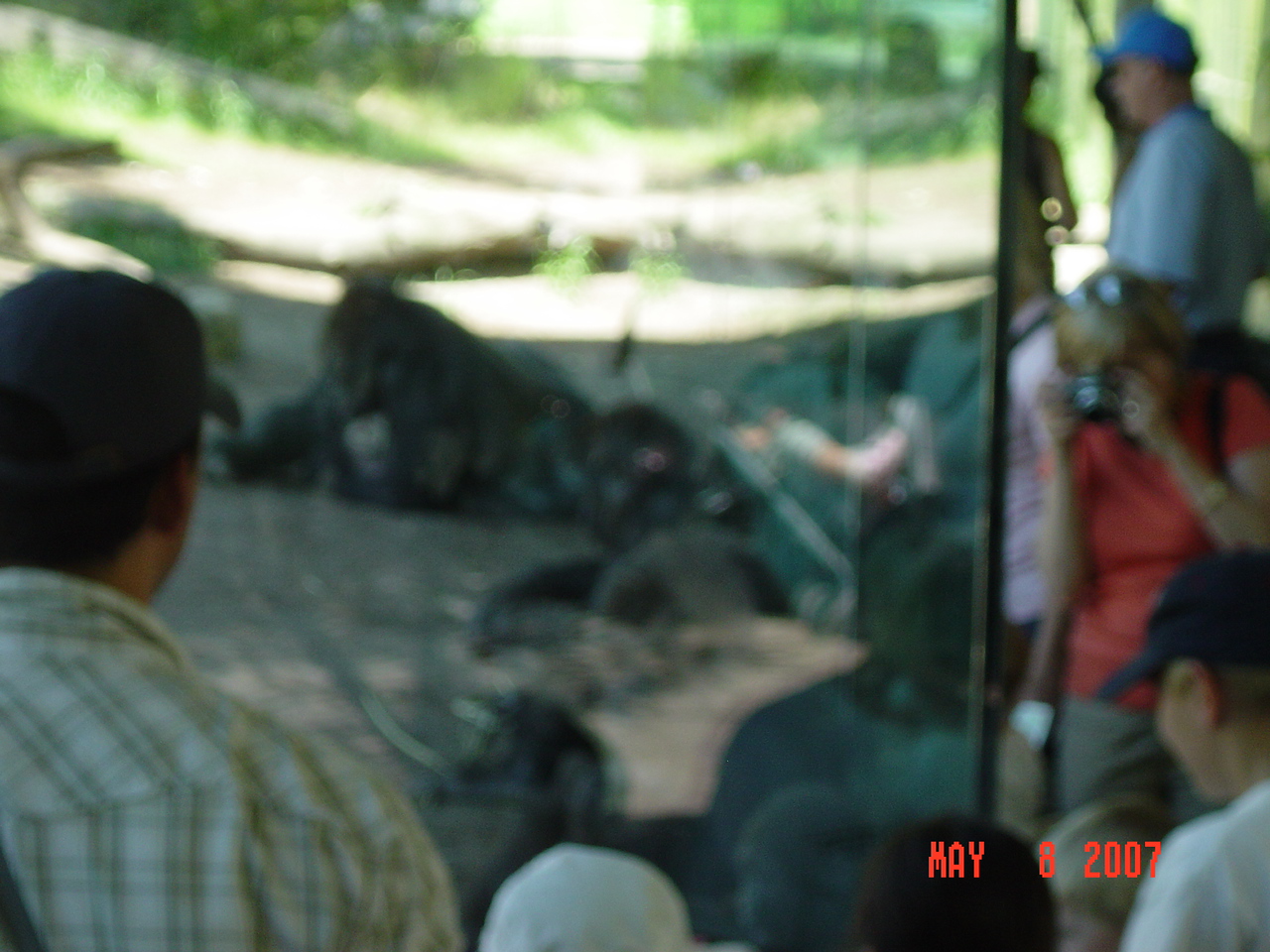This photograph, taken on May 8, 2007, depicts a blurry scene at a zoo where several people, including a woman in a red short-sleeved shirt with a camera, gather around a glass enclosure. They appear to be observing and photographing animals inside, possibly gorillas or other primates, in an environment designed to mimic their natural habitat. The enclosure features plants and rocks, and though the animals are mostly indistinguishable brown shapes, faint reflections in the enclosure might be their eyes. The scene is lit by daylight, and the overall blurriness of the image makes it difficult to discern specific details.